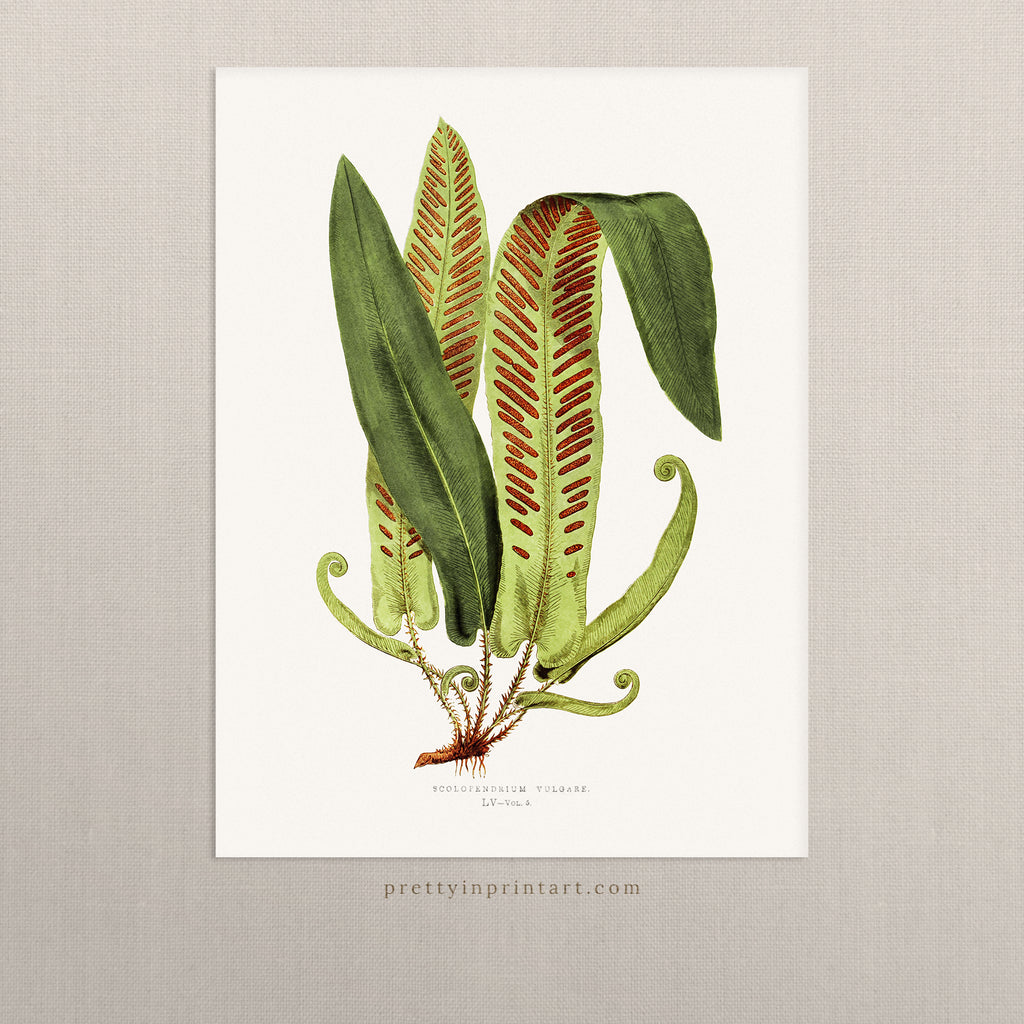The artwork features a detailed and intricate painting of several long, thin, and pointy leaves that are positioned on a white A4 paper background, itself set against a grey backdrop. This composition has the text "prettyinprintart.com" located at the bottom center of the grey area. The painting predominantly uses shades of green and brown, with the leaves varying from dark green to lighter green hues. Some leaves display reddish and orange tones, especially at the base, which resemble spores or small loaves of bread. These leaves are attached to what appears to be a root or tree stalk with stringy, reddish-orange elements. The main leaf, positioned centrally and slightly angled towards the upper left corner, is a dark green, while other leaves bend in various directions, some curling towards the right. The artist's depiction may also include hints of lavender in the background, adding a subtle accent to the overall composition.